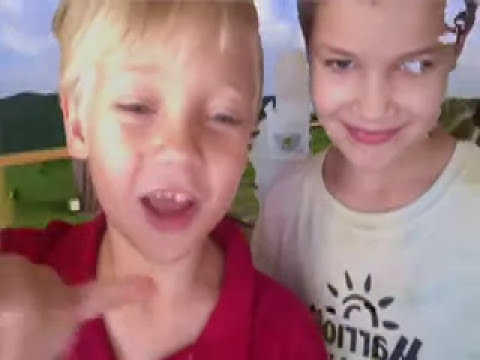In this detailed color photograph in landscape orientation, two smiling children stand side-by-side, dominating the frame from top to bottom. The child on the left is a young boy with straight, blond hair and a gap-toothed smile, seeing as one of his top front teeth is missing. He is wearing a red polo shirt and pointing at the camera with his right hand, a playful gleam in his thin, slightly slit-like eyes. The child on the right, a young girl with dark hair, is wearing a white t-shirt featuring the black text "01776" and a partially visible logo of a half sun. Her eyes are notable as her right eye appears cross-eyed, facing outward while her left eye looks directly at the camera, and part of her face is pixelated, suggesting a photographic distortion or damage. They are posed against a scenic background depicting a green pasture, mountains, and a blue sky adorned with scattered white clouds, offering a sense of serene outdoor beauty.